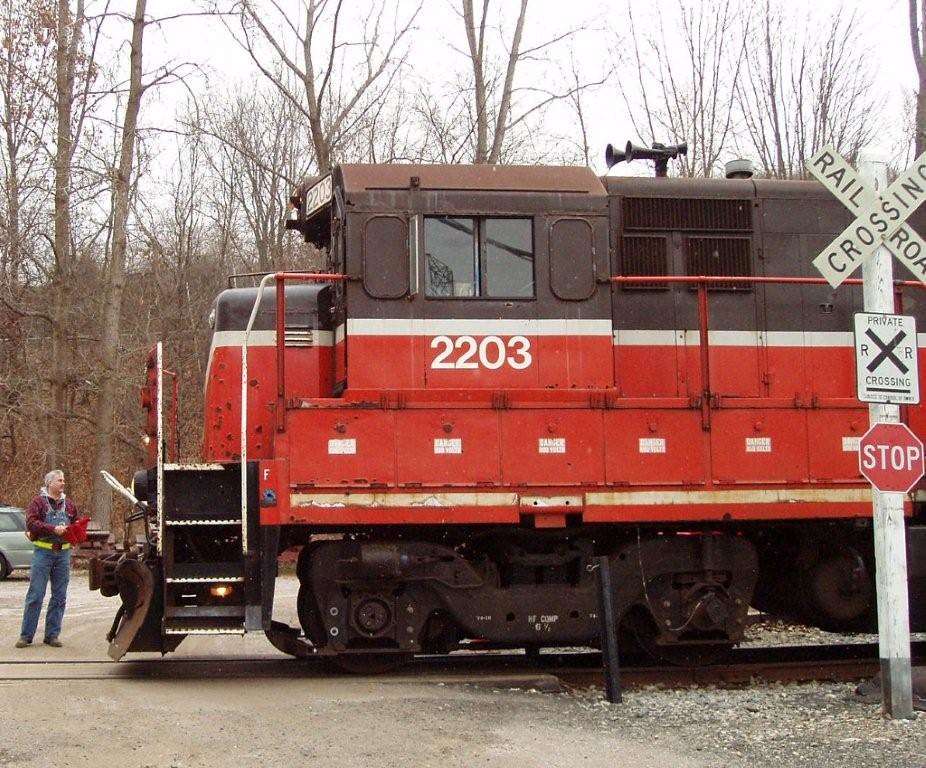The photograph captures the front of a conductor's train car, distinguishable by its dark brown top, red body, and a white stripe near the bottom. Prominently displayed on the side of the train is the number 2203. The train appears to be halted at a railroad crossing, where a tall pole with a stop sign and a private crossing sign stand out on the right side. In front of the train, slightly to the left, an old man is visible. He is dressed in blue jeans and a reddish sweater or perhaps overalls with a red plaid shirt, holding an unidentified red object, possibly a jacket or backpack. The background is dominated by leafless, sparse trees, hinting at a fall or winter setting under a white sky. The front of the train also features a small ladder and black metal wheels, adding to the intricate details of the scene.